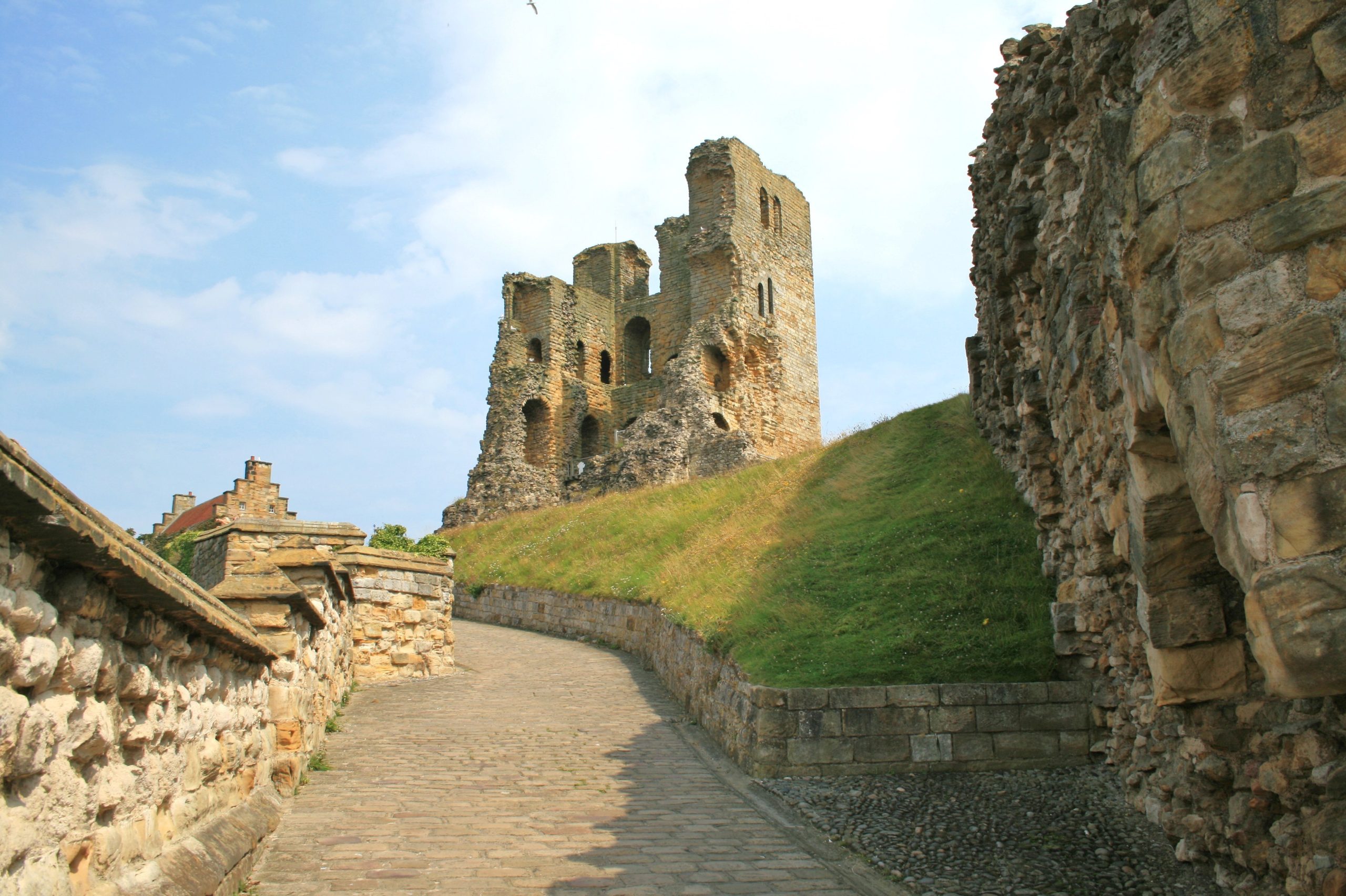The image captures a well-manicured historical site on a bright, sunny day with minimal clouds in the blue sky. At the forefront on the right, a stacked stone wall of various types of stones borders a hilly grassy area, flanked by a light brown brick pathway. A shorter brick wall is also visible on the left. The path leads up to an impressive but decayed historical building made of light brown or gray stone, situated on an elevated part of a hill or mountain. This structure, likely several centuries to a thousand years old, stands three to four stories tall and lacks a roof. Many walls are missing, revealing cutouts for windows. In the background, another historical building appears more intact, contrasting with the ruins in the foreground.